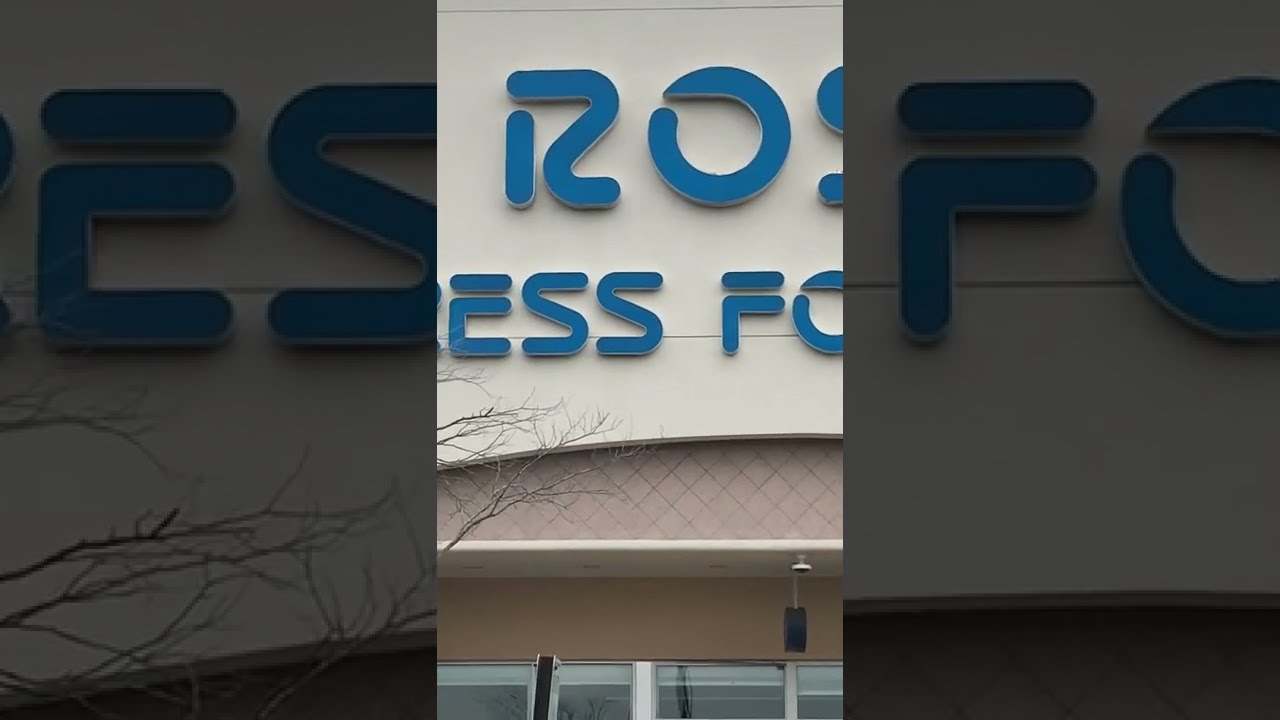The image depicts a "Ross Dress for Less" store sign, segmented into three parts with distinct lighting effects. The left and right thirds are shadowed, showcasing the letters "E" and "S" on the left, and "F" and "O" for "for" on the right, all in dark blue against a beige background. The central section is brighter, prominently displaying the letters "R," "O" at the top, and "E," "S," "S," "F," "O" below. This triptych zoom-in emphasizes different parts of the store's sign, revealing a bit of the business's architecture and a tree in the foreground. The colors visible include off-white, blue, tan, black, and silver, and the image appears to be a mobile screenshot from an app like TikTok or Instagram.